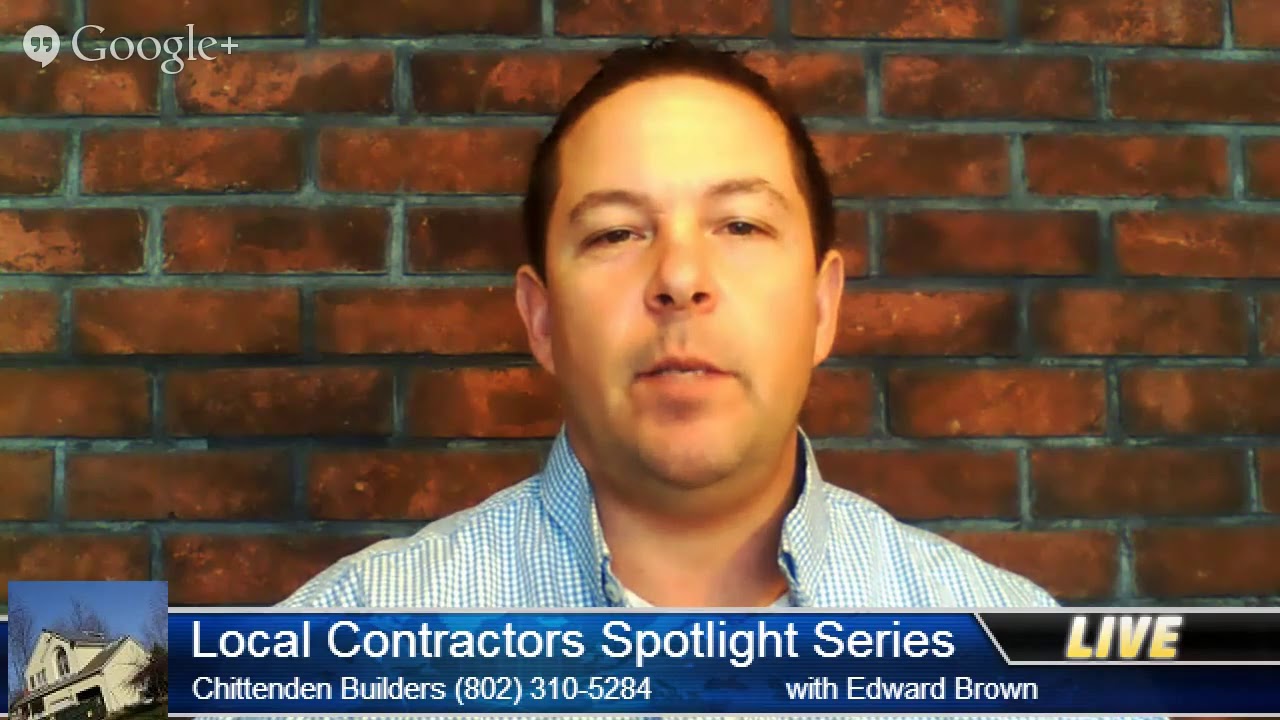Screenshot from a Google Plus Live broadcast featuring Edward Braun, who is discussing his contractor business, Chittenden Builders. Edward, wearing a cool blue checkered shirt with a white undershirt, is standing against a red brick wall, appearing engaged and mid-speech while offering insights about his services. The upper left corner of the image features the Google Plus logo, indicating the platform for the live session. A small thumbnail of a house, possibly one Edward built, is displayed in the lower-left corner. The lower-third of the screen contains a blue newsreel strip with white text that reads, "Local Contractors Spotlight Series, Chittenden Builders, 802-310-5284, With Edward Braun," highlighting Edward and his business. A yellow, italicized "live" text is noticeable in the lower right corner, emphasizing the real-time nature of the broadcast.